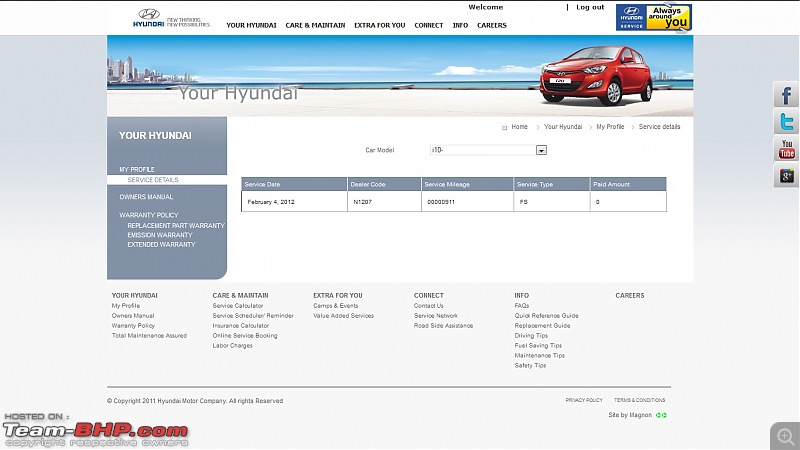This is a detailed and organized caption for the image described:

---

This webpage belongs to Hyundai, displaying their legal logo in a grey color. The header section includes the Hyundai tagline "Always around you" and navigation options such as "Welcome" and "Log Out," all laid out on a white background with black text. Below the header, there is a long image featuring a vibrant blue sky and a red Hyundai car positioned on a light tan cement surface, with a cityscape in the background. The text "Your Hyundai" appears on the left side of the image.

The left sidebar of the webpage is grey and includes various links like "My Profile," "Service Detail," "Owner's Manual," "Warranty Policy," "Replacement Parts Warranty," "EV & Sun Warranty," and "Extended Warranty." The main content area is white, focusing on the "Service Detail" section, which is currently open. Displayed details include:
- Date: February 4th, 2012
- Service Order Number: N1207
- Service Mileage: 00000911
- Service Type: Number 5
- Paid Amount: 0

The design uses a mix of colors and sections to organize information clearly for Hyundai users.